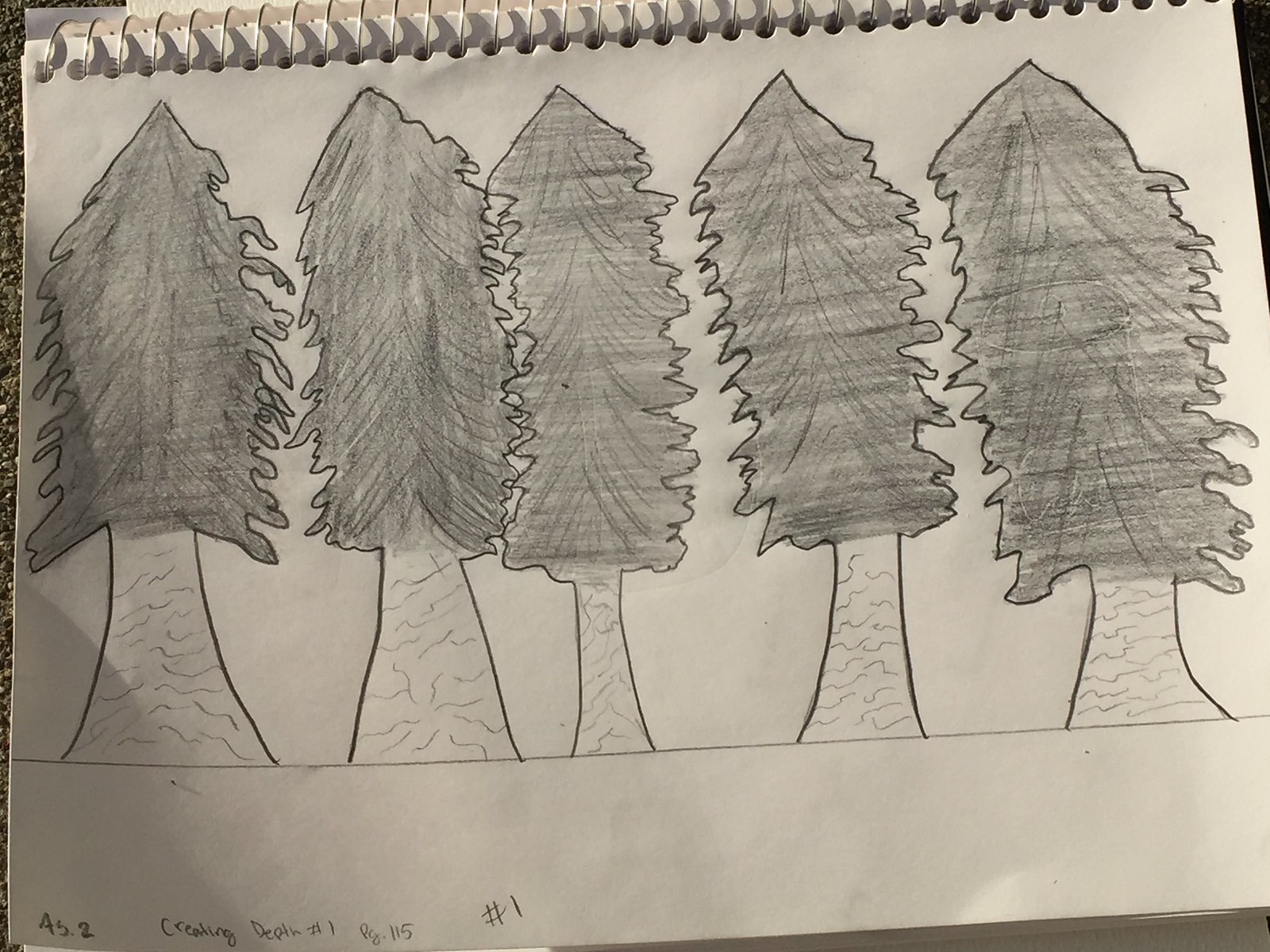A spiral notebook with an off-white page is depicted horizontally, showing the silver spiral binding at the top. The page features a detailed pencil sketch of five pine trees of varying sizes, outlined in black and filled with shaded lines to represent texture. Each tree is drawn with wide, triangular bases and small trunks. A horizontal line near the bottom of the page acts as the ground for the trees, extending across the entire width of the paper. The middle two trees slightly overlap with their branches. In the bottom left corner, the page has some indistinct writing including numbers like "45.2", "115", and possibly "creating depth number 1". The image background shows some black elements, suggesting it is sitting on a black surface.